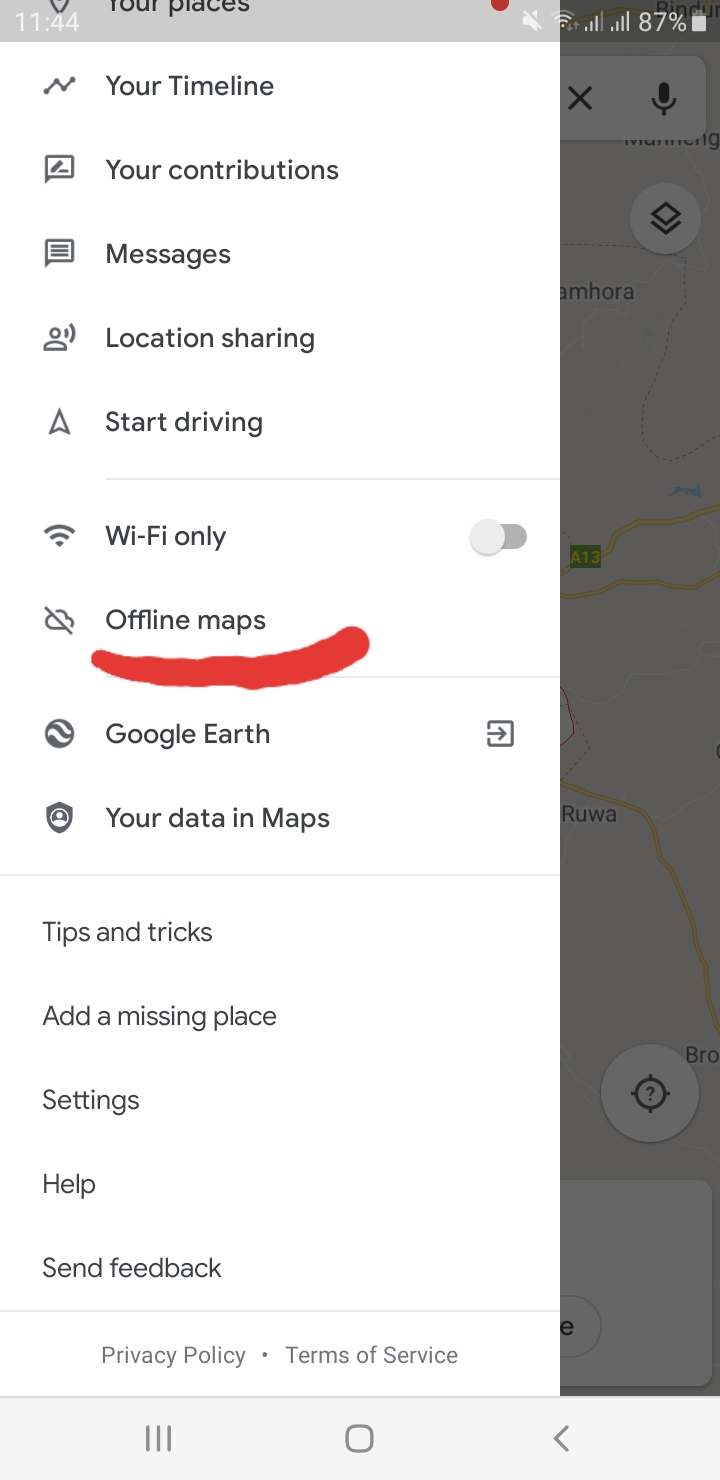The image displays a smartphone screen showcasing an admin panel for an application that appears to be Google Earth. The user interface consists of a grayed-out map in the background, with visible yellow lines and highway markings, partially obscured by an overlay panel that has slid in from the left. The current time displayed is 11:44, the phone is in silent mode, and full Wi-Fi connectivity is indicated, along with two signal bars showing 3 out of 4 and 4 out of 4 respectively. The battery level is at 87%.

On the overlay panel, a series of gray icons are positioned to the left of the corresponding text options. The detailed panel includes:
1. A line graph icon next to "Your Timeline"
2. A speech bubble icon beside "Your Contributions"
3. Another speech bubble icon next to "Messages"
4. A person speaking icon labeled "Location Sharing"
5. A paper airplane icon labeled "Start Driving" (depicted as a navigation arrow)
6. A Wi-Fi signal icon beside "Wi-Fi only," which is currently toggled off
7. A cloud with a slash icon labeled "Offline Map," beneath which there is a playful, red scribble resembling a smiley face
8. A globe icon labeled "Google Earth"
9. A shield icon beside "Your Data in Maps"

Further down the panel, without accompanying icons, are the options "Tips and Tricks," "Add a Missing Place," "Settings," "Help," and "Send Feedback." At the very bottom, there are text links for "Privacy Policy," indicated by a dot separator, and "Terms of Service." The bottom of the screen features a standard navigation bar against a white background.

This intricate depiction provides a comprehensive view of the app’s overlay panel, showcasing various functional options typically available to the user.